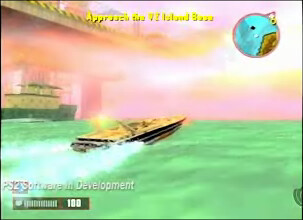The image is a digital art screencap from a PS2-era video game interface. At the top left, there's a mini-map displaying an ocean and surrounding land with the player's position, while the main objective, written in yellow text at the top center, instructs to "approach the island boss" (though this text is somewhat difficult to decipher). Dominating the scene, the main visual features a small speedboat cutting through blue-green water, leaving turbulent waves in its wake. To the far left, there's a larger commercial boat near what seems to be an oil rig or a large building structure. In the foggy background, a bridge is faintly visible. The bottom of the screen has a black rectangle displaying a health meter marked "100" and the phrase "PS2 software in development" indicating the game's developmental status. The image is framed against a black background, completing the retro video game aesthetic.